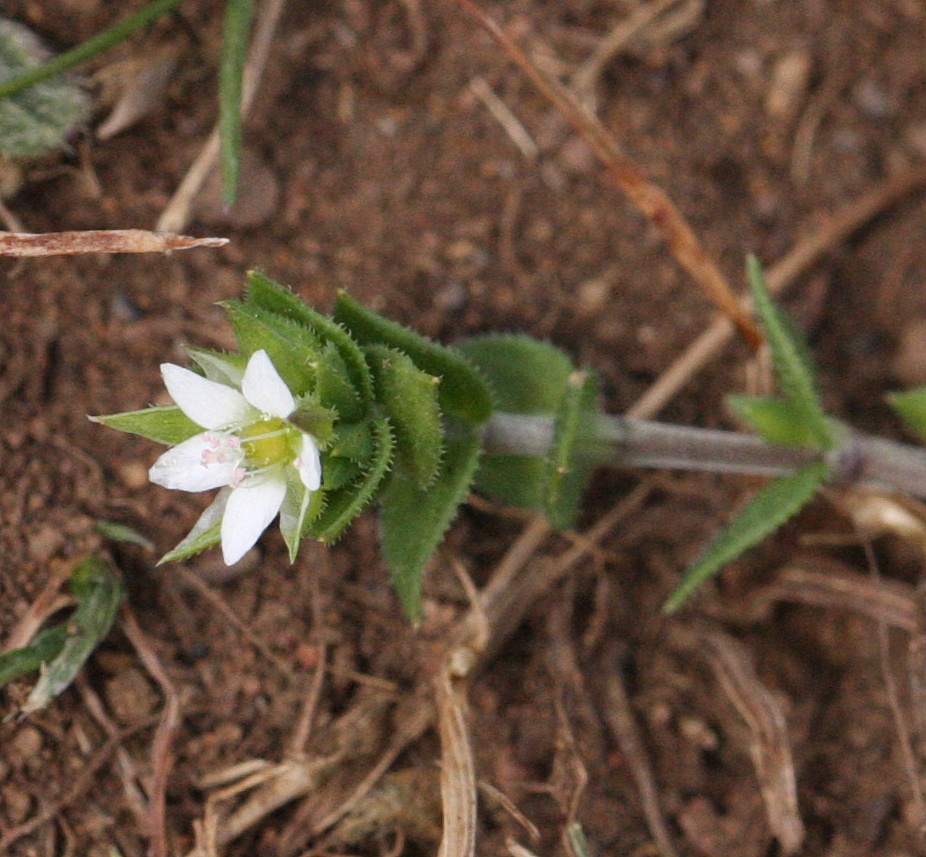This image showcases a vivid scene of a groundrunner plant prominently displayed against a backdrop of dark brown dirt scattered with mulching. The plant, primarily shooting from right to left, features a brown stem, which is covered in a fine white fuzz. The stem supports several arrow-shaped, vivid grass-green leaves, each adorned with tiny, spike-like thorns along their edges. These staggered leaves increase in density closer to the top, where they surround a strikingly detailed white flower. The six arrow-shaped petals of the flower frame a center composed of an off-yellow stamen and pistil with subtle pink and white tips. The plant's new growth appears small compared to its branched stalk, which exhibits a distinct round purple hue, in contrast to the green leaves. The ground beneath the plant is mostly brown and blurry, drawing focus to the plant itself, which appears to be in the early stages of growth with some sections of the branch still bare of leaves.